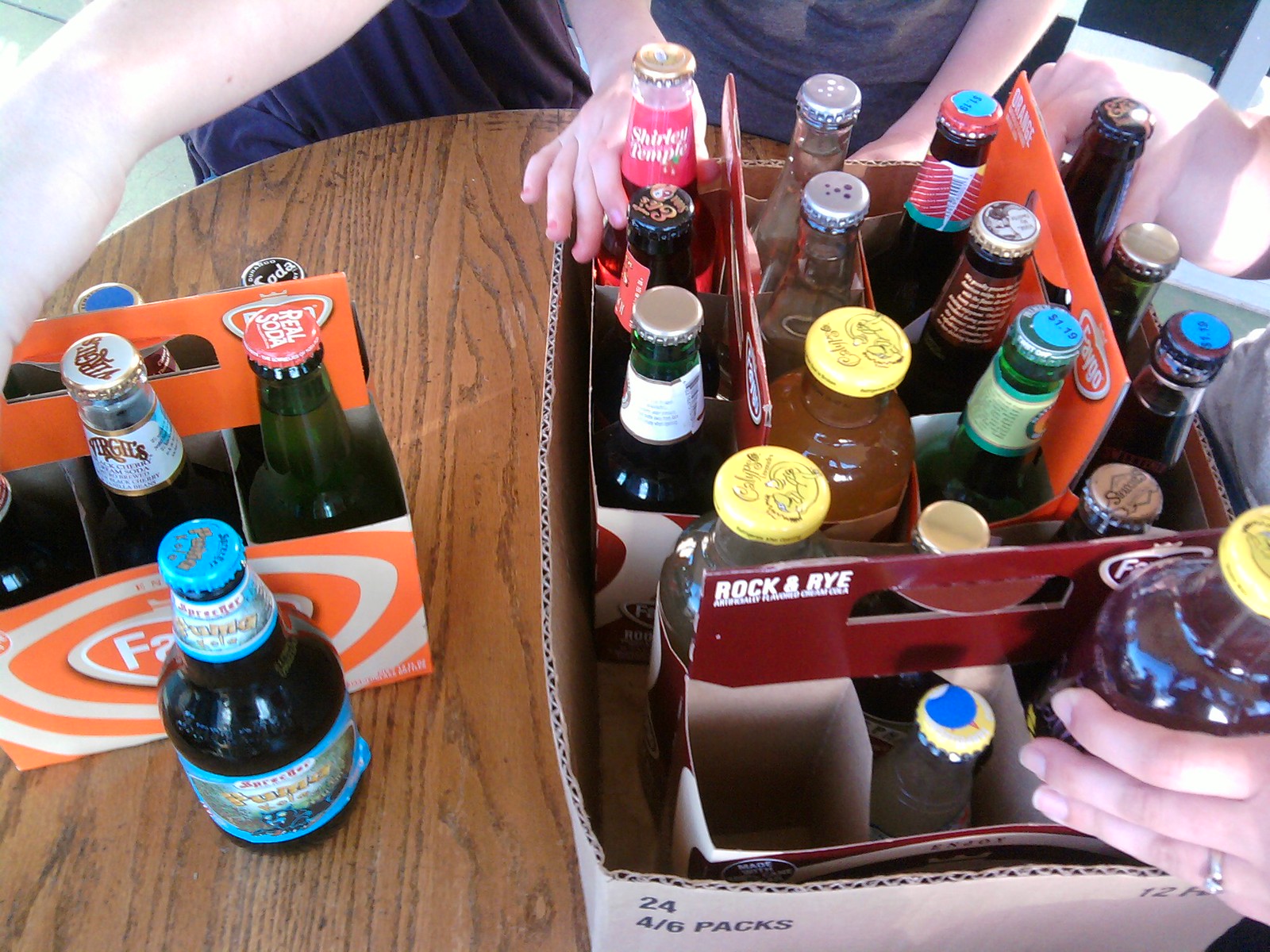The image showcases a scene of a few people, mostly identifiable by their torsos and hands, gathered around a round, light brown wooden table. The focus is on a variety of drinks organized in multiple carrying cases. There are more than 10 glass bottles of different shapes and colors, marked with tags in blue, maroon, and yellow. Some of the bottles have the slender shape typical of beer bottles and have different colored tops, while others are wider with screw-on caps. Two of the smaller bottles, suggesting they require a bottle opener, stand out among the collection. The drinks are neatly placed in cardboard carriers with cut-out handles for easy transportation. Additionally, the layout includes another cardboard box filled with bottles and an orange six-pack container holding yet more drinks, along with one loose bottle on the table. The table appears cluttered with these various containers, and two individuals in black shirts are seen organizing the assortment of drinks.